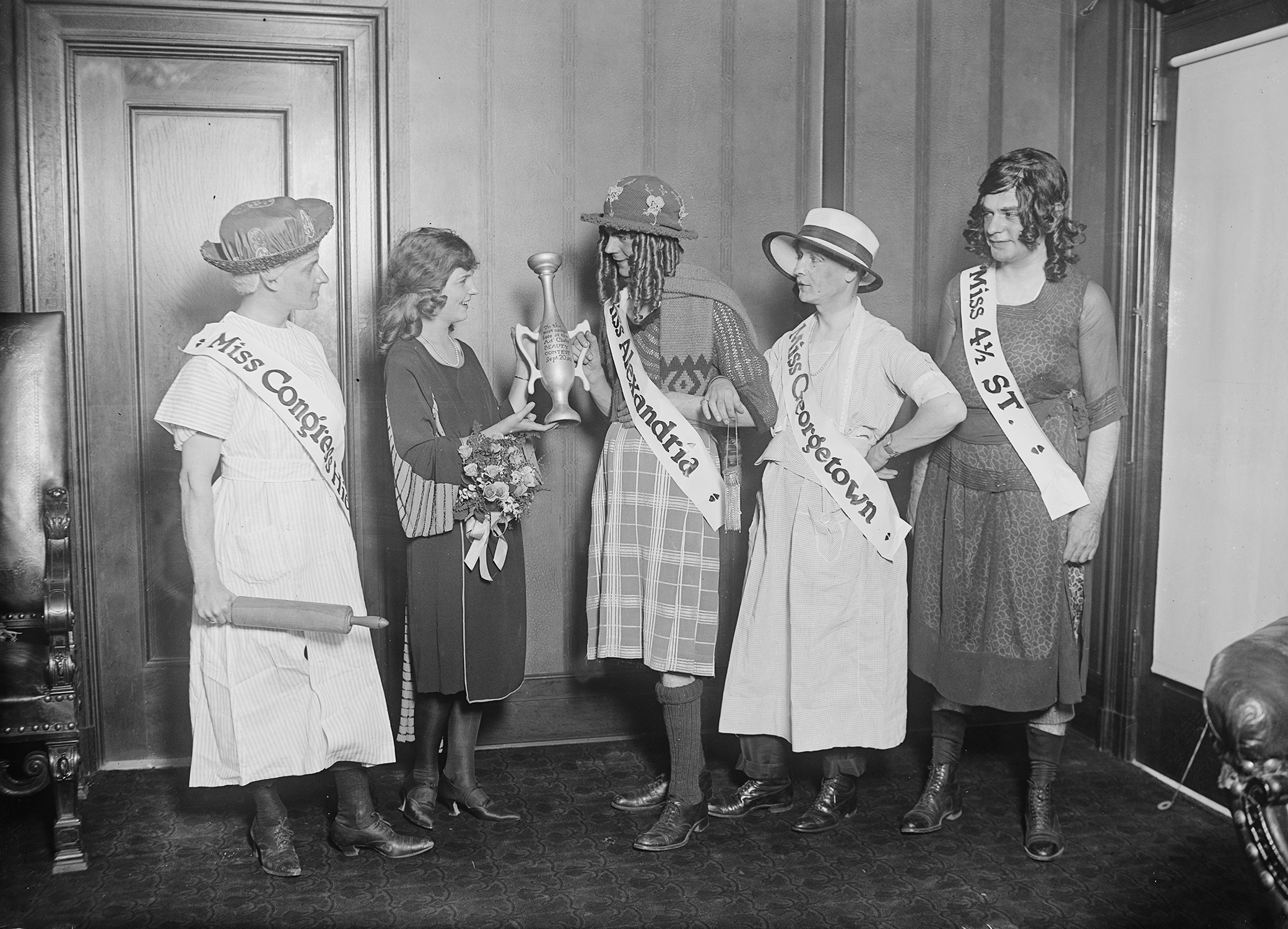This black-and-white photo, likely from the 1930s to 1950s, captures a humorous mock awards ceremony for a beauty pageant. In the center, a woman is handing a vase trophy to a man dressed as a woman, identified by the sash reading "Miss Alexandria." Four other men, also dressed as women, stand around them in various dresses, some white, some plaid, and others with different textures. Their sashes read "Miss Four and a Half Street," "Miss Georgetown," and "Miss Congress." Notably, one person in the scene is holding a rolling pin, adding to the comical nature of the event. All participants’ attention is focused on the award presentation.